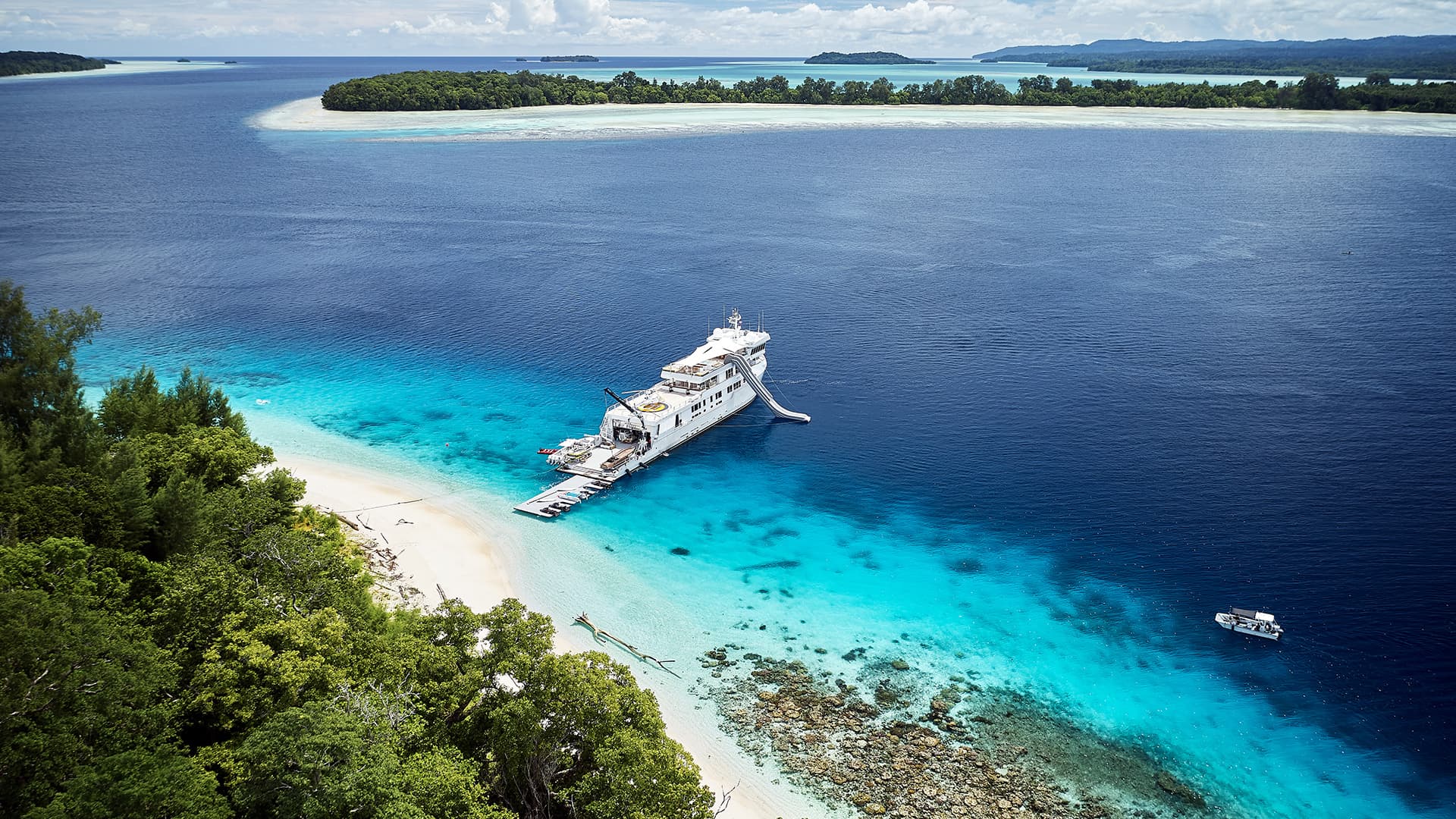The image appears to be an aerial photograph showcasing a picturesque coastal scene. Dominating the lower left side of the image is a stretch of white sandy beach, bordered by lush green trees. Just off the shore, a large white yacht is prominently featured, partially beached with its stern extending a white plank down onto the sand. The surrounding waters exhibit a gradient of blues, from light turquoise near the beach to deeper shades further out. In the lower right corner, a smaller white boat approaches the larger yacht. The upper portion of the image reveals additional landmasses and islands with dense green foliage and more pristine beaches. The bright daytime sky is adorned with scattered white clouds, enhancing the overall serene and idyllic atmosphere.